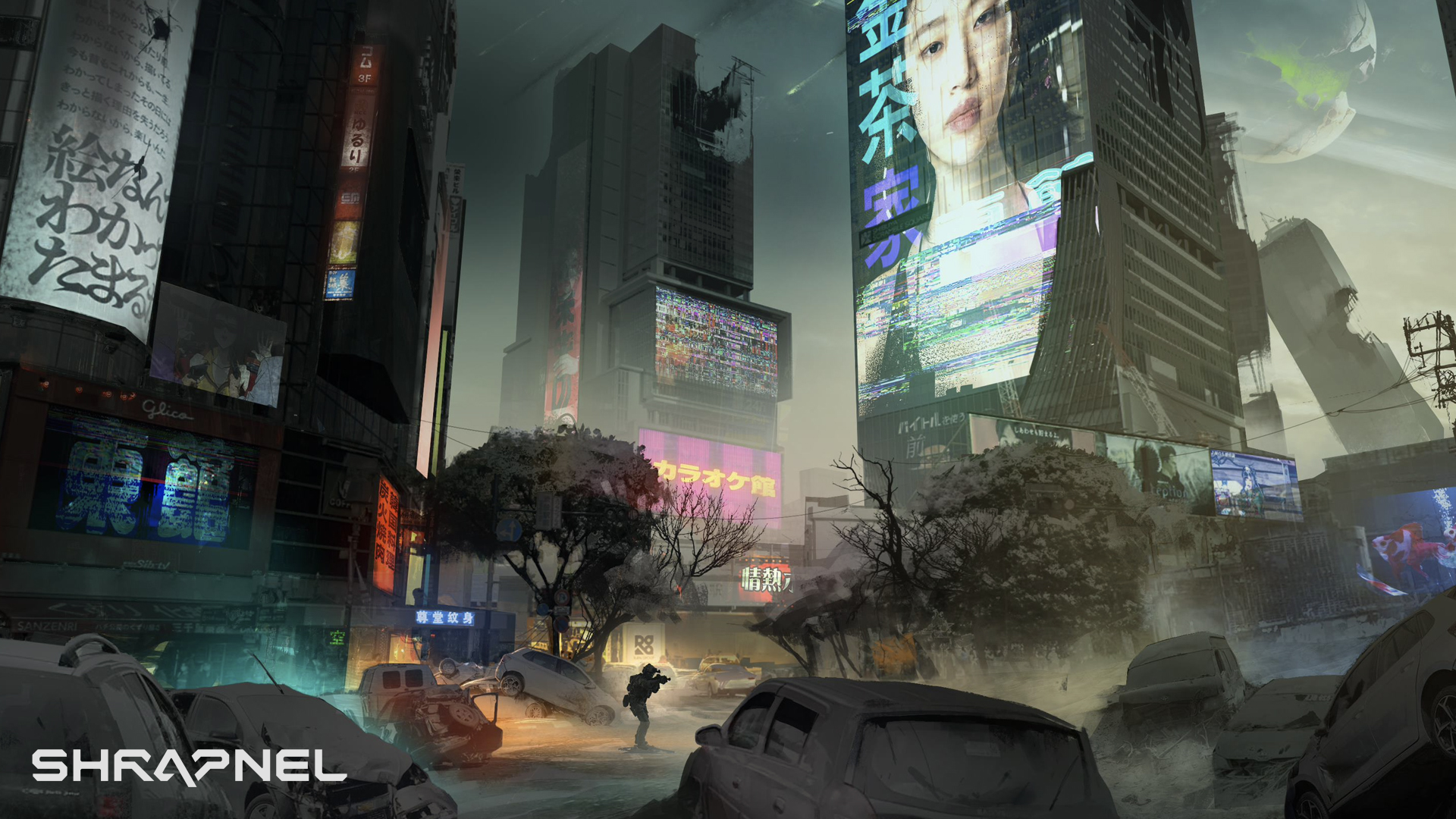This image depicts a highly detailed, AI-generated, dystopian cityscape, possibly inspired by downtown Japan or another oriental metropolis. The scene is marked by significant destruction, with several skyscrapers showing large holes as if they have been hit by explosions, and the streets are littered with destroyed cars, some overturned or upended. In the bottom left corner, there is a white watermark text that reads "shrapnel" in a futuristic font. 

A military figure, dressed in black and holding a gun, stands in silhouette among the wreckage, facing a tree that has lost much of its foliage. The tree's black branches stretch up into the hazy gray sky, which veils the scene in a polluted, smoky atmosphere with a greenish tint. In contrast, there are blue luminescent lights emanating from the car headlights and buildings, contributing to the eerie glow of the environment. 

Large billboards with oriental script and images of women can be seen on the skyscrapers' large, TV-like screens, adding to the apocalyptic essence of the image. A prominent advertisement featuring an Asian lady with accompanying Japanese characters is particularly notable. The atmosphere is further disturbed by the presence of ash or snow coating the trees and the debris-laden streets, hinting at the remnants of a catastrophic event. To complete the apocalyptic ambiance, a large moon or planet looms in the upper right part of the sky, overlooking the devastation below.